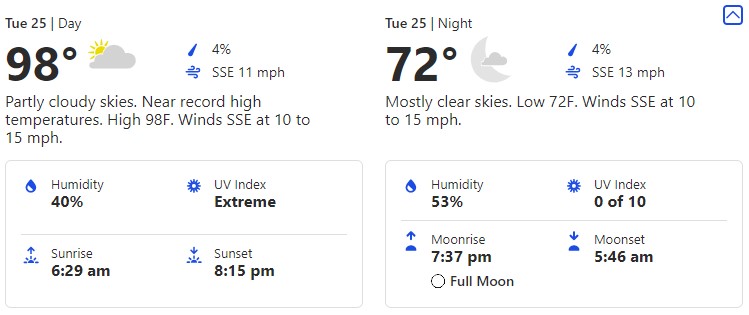This weather app screenshot details the forecast for Tuesday, the 25th. During the day, temperatures are expected to reach a near-record high of 98°F. The sky will be mostly cloudy with a 4% chance of precipitation. Winds are projected to move from the south-southeast at 11 mph. The detailed forecast indicates that the day will be partly cloudy with high temperatures near 98°F and winds ranging between 10 to 15 mph from the south-southeast.

Additional daily metrics are displayed in a grid format:
- Top left: Humidity at 40%
- Top right: UV Index rated as ‘Extreme’
- Bottom left: Sunrise at 6:29 AM
- Bottom right: Sunset at 8:15 PM

The nighttime forecast predicts mostly clear skies with a low of 72°F, and the wind continuing from the south-southeast at 10 to 15 mph with a 4% chance of precipitation. Nighttime humidity rises to 53%. Moonrise is at 7:37 PM, and moonset occurs at 5:46 AM, with a UV index of 0 out of 10.